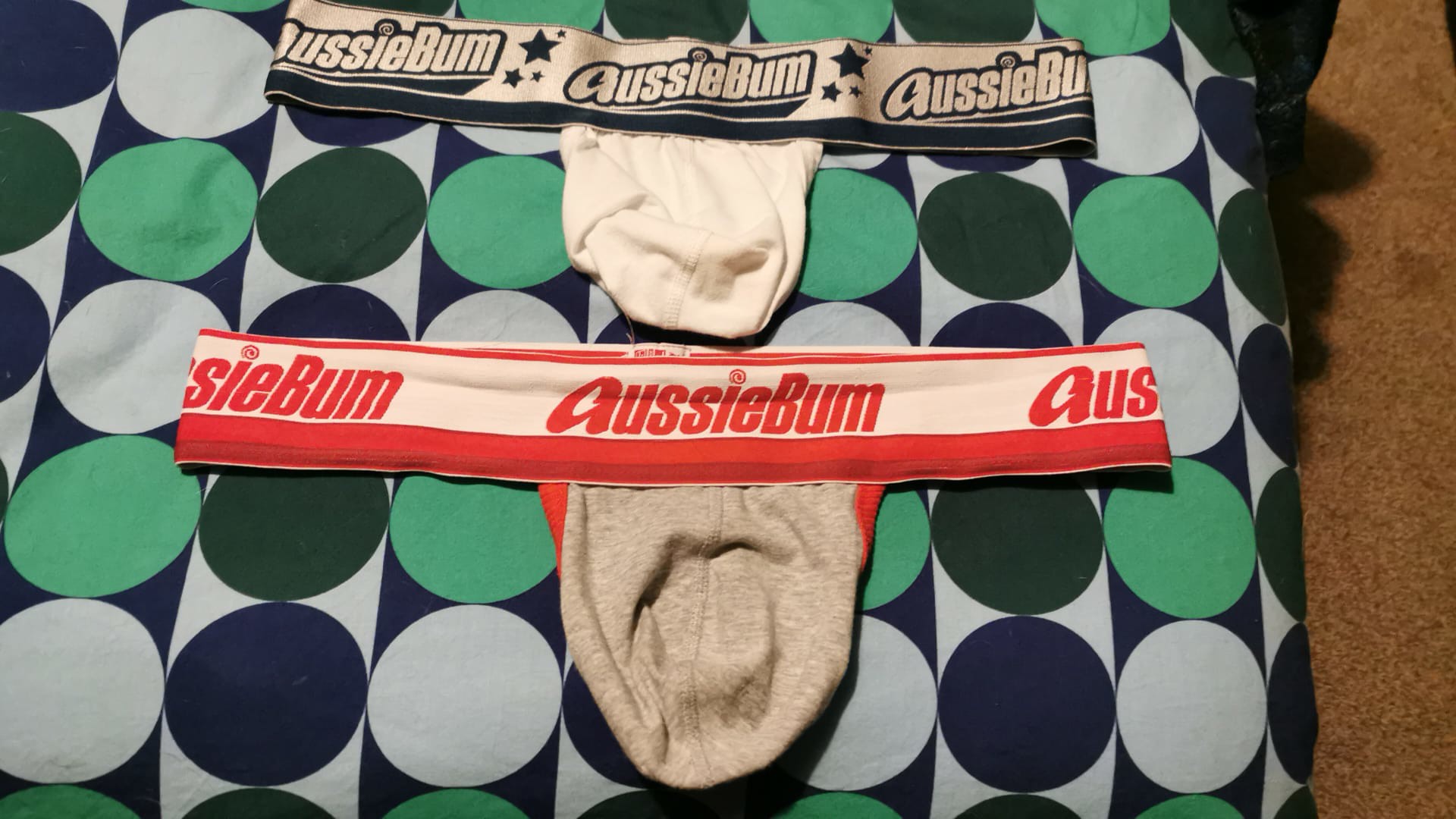This color photograph displays two pairs of men's jockstraps arranged on a bedspread featuring a black background with white and green polka dots and circles. The image, taken in landscape orientation, shows the top jockstrap prominently featuring a white waistband with black trim, emblazoned with the brand name "AussieBum" written three times in black, accompanied by alternating large and small blue stars. This jockstrap pouch is white. The jockstrap beneath it sports a similar design, with a red and white waistband also branded with "AussieBum" in red letters, though this band lacks stars. Its pouch is brown. The detailed backdrop and the contrasting jockstrap designs create a visually engaging composition with a focus on the branding and color patterns.